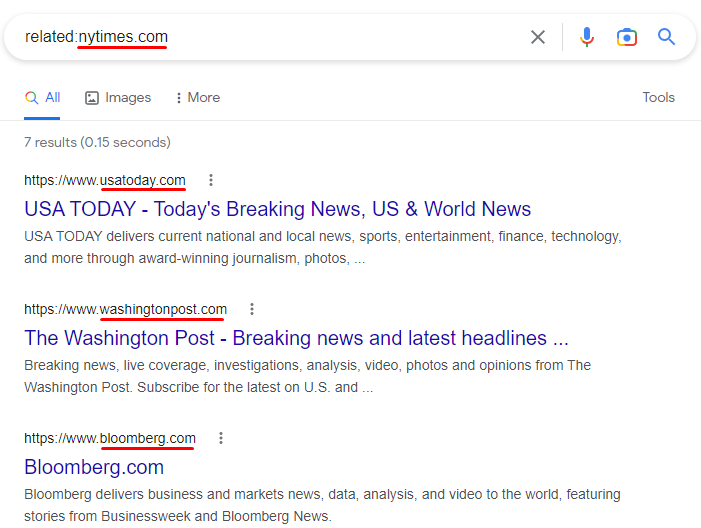A detailed screenshot of a Google search is showcased in this image. The search query entered into the search bar is "related:NYTimes.com" with no spaces following the colon. Notably, "NYTimes.com" is highlighted with a red underline. The search results are displayed below the search bar, and it is evident that they do not include the New York Times.

The top result is from USA Today, reading "USA Today: Today's Breaking News, U.S. and World News." The second result is from The Washington Post, labeled "The Washington Post: Breaking News and Latest Headlines." The third result is from Bloomberg, succinctly titled "BloombergDark.com." Each of these web addresses is similarly underlined in red, indicating that they did not match the expected NYTimes source.

At the top of the results section, Google notes that there are "7 results (0.15 seconds)." Additional options for refining the search appear along this line, including buttons for viewing images, accessing more search results, and employing further tools, with the "Tools" option positioned on the far right.